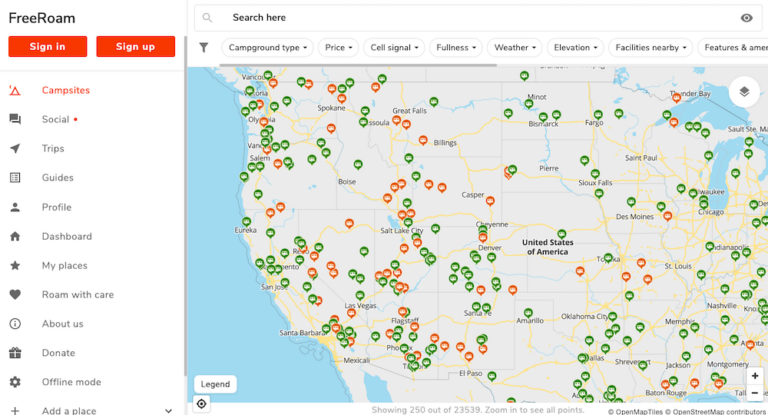The image features a detailed map of the United States displayed on a website, covering the region from the west coast up to approximately Michigan, and cutting off near the Great Lakes. The map itself presents the US in a white background, scattered with numerous green and red markers resembling location pins. These pins are circular with small arrows at the bottom, indicating campsite locations.

Above the map, there is a search bar labeled "Search here." Below the search bar, a series of filter menus are displayed, including options for "Campground Type," "Price," "Cell Signal," "Fullness," "Weather," "Elevation," "Facilities Nearby," and "Features and Amenities."

On the left side, a vertical menu titled "FreeRoam" is visible. This menu includes two orange buttons for "Sign In" and "Sign Up," and various categories such as "Campsites," "Social," "Trips," "Guides," "Profile," "Dashboard," "My Places," "Roam with Care," "About Us," "Donate," "Offline Mode," and "Add a Place."

The overall impression suggests that this map is an interactive tool for exploring and identifying campgrounds across the United States, with additional features for planning and managing camping trips.